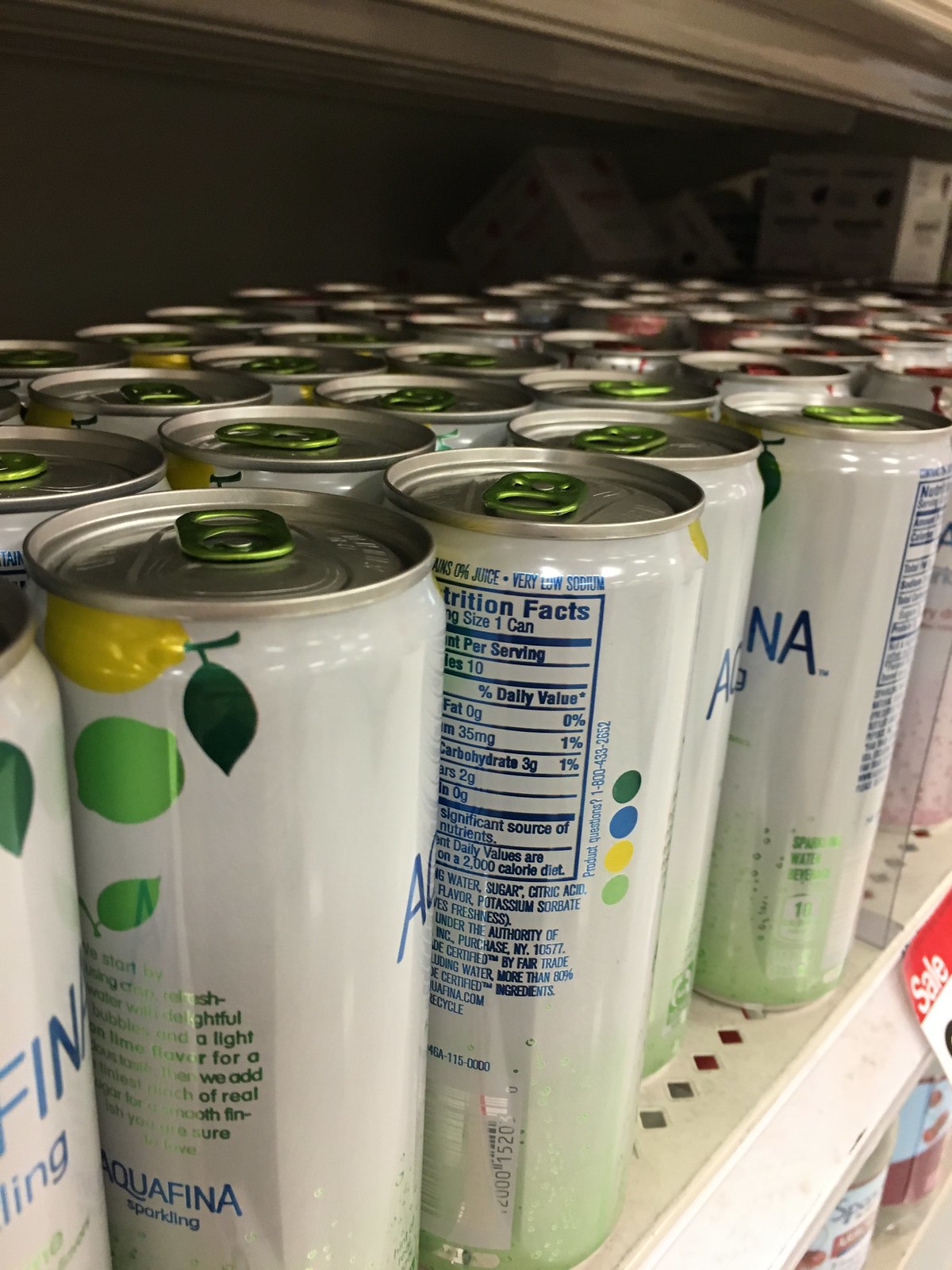The image is a close-up taken in a grocery or department store, showcasing approximately 20 cylindrical cans of Aqua Fetus Sparkling drink. Each can features a sleek design with a white and silver color scheme that gradually fades into green towards the bottom. The tops of the cans are fitted with green pop tops, though some cans in the background have red pop tops. A detailed nutrition facts label is visible on the back of the cans, accompanied by green writing. The arrangement and uniformity of the cans highlight the product's bright and refreshing appearance.